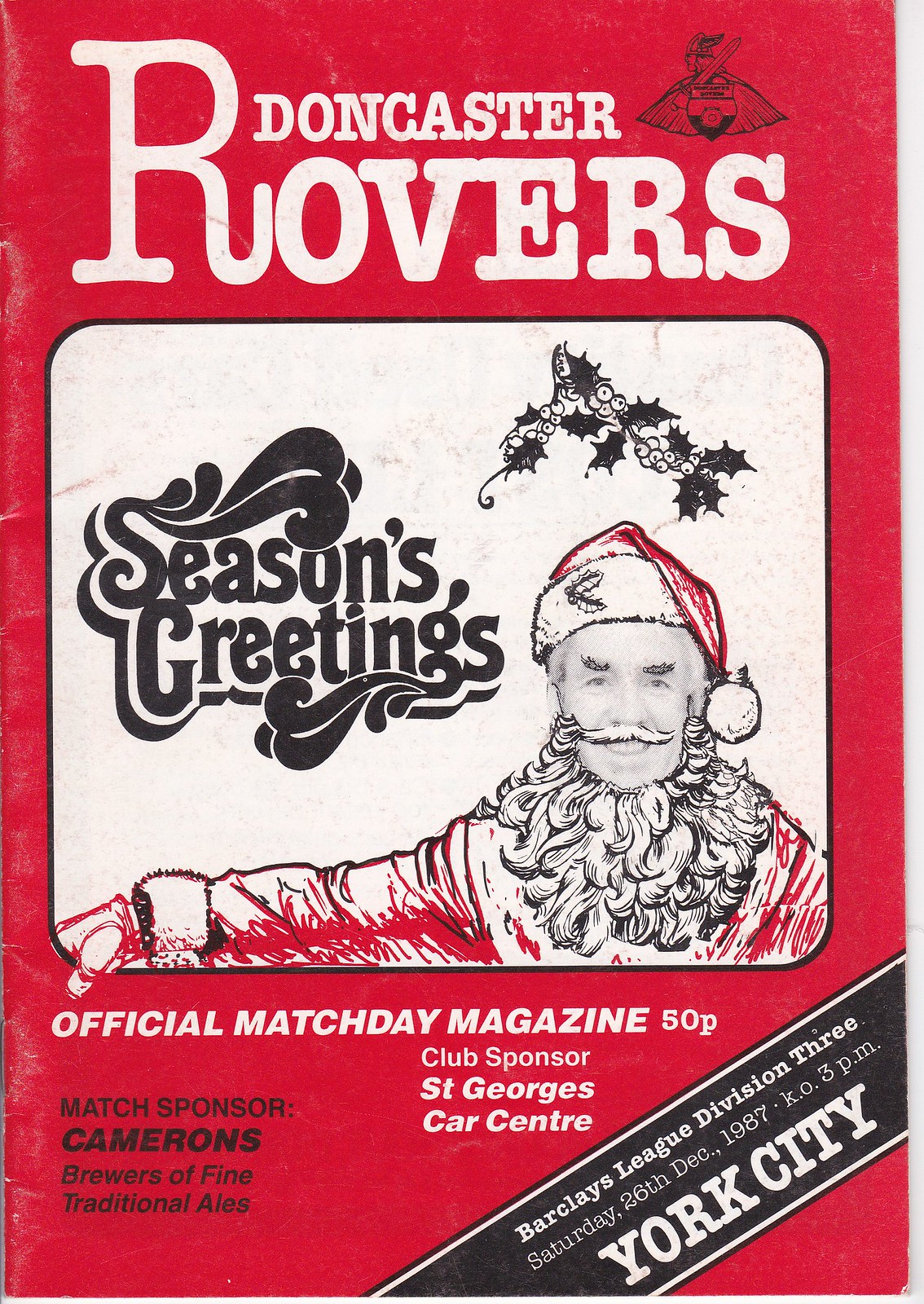This image is a festive poster for the Doncaster Rovers soccer team's official match day magazine, themed around Christmas. At the center of the image is a person dressed in a Santa costume, with a distinguishing detail of their beard not fully covering their chin. Santa's right hand is extended outward, and holly is positioned above him. To the top right of Santa, there is the Doncaster Rovers team logo. The background is predominantly red, enhancing the holiday theme, with the white and black of Santa's beard and hat, matching the white text on the poster. The accompanying text reads "Doncaster Rovers Seasons Greetings," along with promotional information including "Official Match Day Magazine," "Club Sponsor: St. George Car Center," and "Match Sponsor: Camerons Brewers of Fine Traditional Ale." Additional details specify it is related to a soccer match played in the Barclays Division III against York City. The aesthetic of the poster, combining red and white with festive Christmas elements, clearly indicates it is designed for a soccer event around the holiday season.